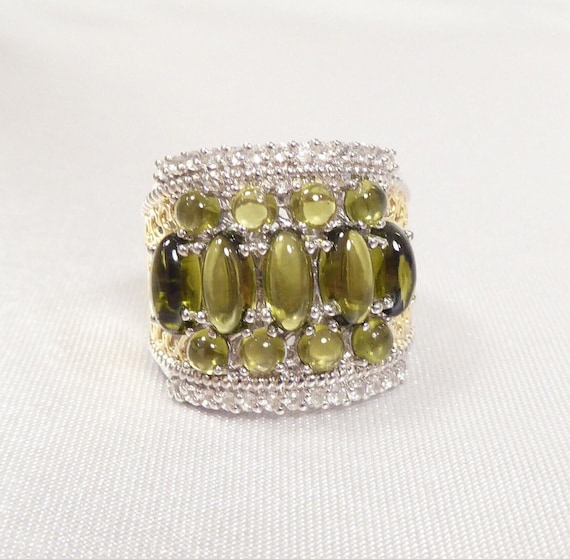The image is a rectangular photograph approximately four inches by four inches, featuring a large, thick ring positioned on its side in the center. The background is primarily white, blurring slightly towards the top, and transitions to a blue and white fabric with horizontal or vertical raised ridges or threads, potentially a napkin. The ring itself is intricately designed, adorned with rows of white-looking stones set in silver at both the top and bottom edges. Between these, there are smaller round olive green gemstones, with four on top and four on the bottom. The center band of the ring showcases five larger, oval-shaped olive green gemstones, resembling the appearance of fish oil pills. Both the smaller and larger stones contribute to a detailed and striking visual symmetry.